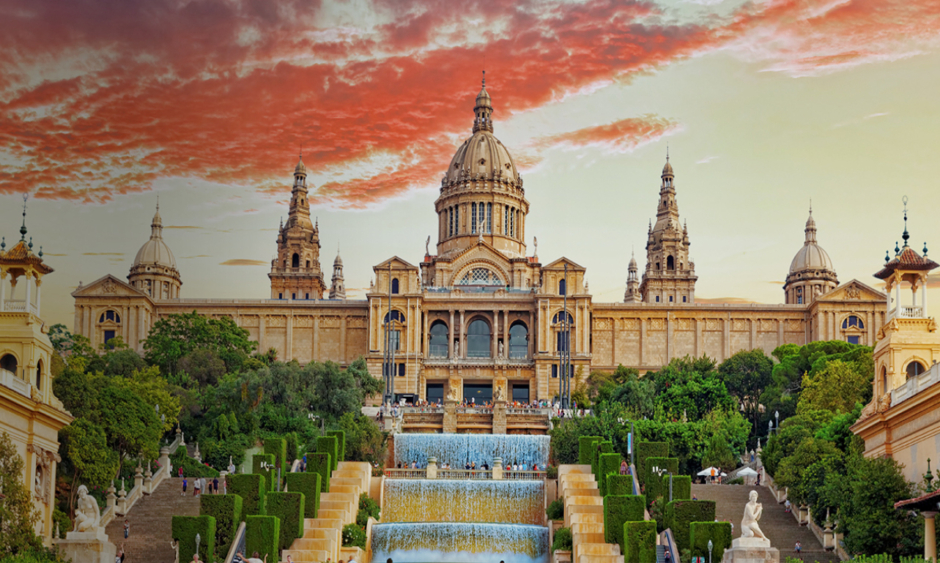The photograph captures a grand, palace-like building perched atop a hill, bathed in the warm hues of sunset, with the sky painted in shades of orange and yellow. This rectangular edifice, reminiscent of a classic palace, features a facade adorned with multiple glass-pane archways and is crowned by several domes and towers. In the center, a prominent dome with a spire catches the eye, while other towers rise to graceful points.

Leading up to the building are two sets of stairs, situated on the bottom left and right, each flanked by short brown stone railings and bordered by meticulously manicured green square-shaped bushes. These stairways converge towards the center, framing a multi-tiered waterfall-like fountain that cascades elegantly from the palace's upper balcony, where people can be seen gazing down at the spectacle. Marble statues of naked women stand guard at the base of the steps, enhancing the scene's classical elegance. The entire scene is harmoniously nestled against a hillside, enriched by the vibrant, sunset-streaked sky, lending an enchanting atmosphere to this architectural marvel.